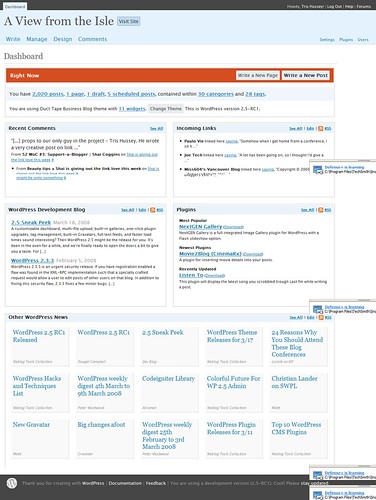A detailed screenshot of a computer screen is depicted in the image. A black border runs along the top. On the left, an open tab is labeled "Dashboard," while a "Log Out" button is situated to the right. The screen features a light blue section prominently displaying the title "A View from the Aisle," alongside a button labeled "Visit Site."

Below this, a navigation bar includes options such as "Write," "Manage," "Design," and "Comments." The central portion of the screen shows a white area headed "Dashboard" and a red-bordered section with a prompt that reads "Write Now." To the right, it offers options to "Write a New Page" or "Write a New Post."

The middle of the screen contains four rectangular sections: the top left being "Recent Comments," the top right "WordPress Development Blog," the bottom left "Incoming Links," and the bottom right seemingly labeled "Pledges." Additionally, at the very bottom, a section titled "Other WordPress News" displays a grid of squares organized in three horizontal rows, each consisting of five boxes.